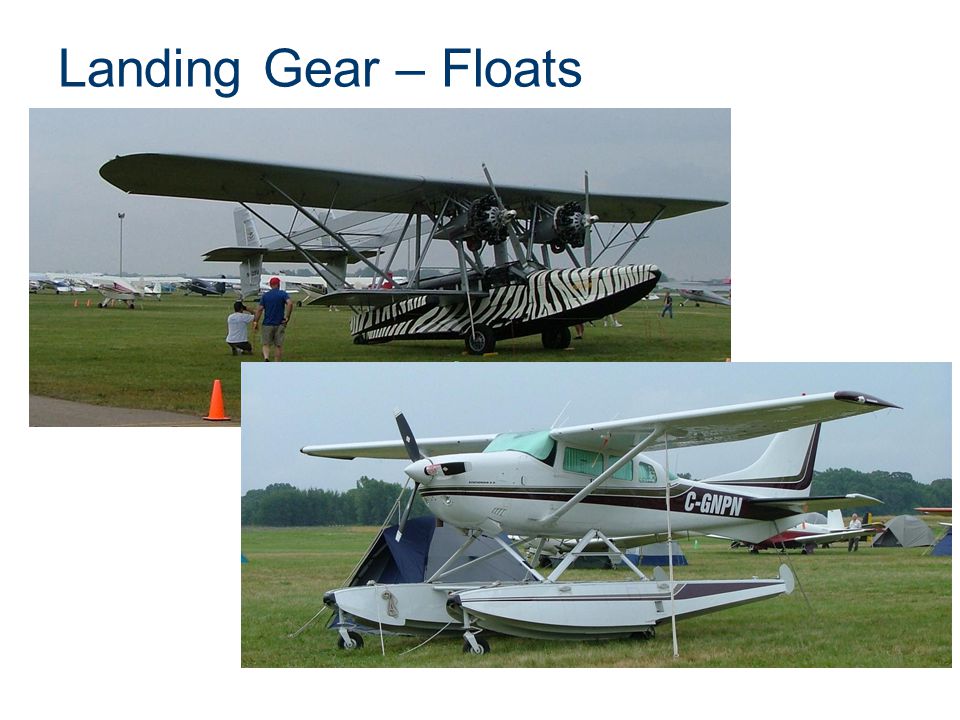The image is divided into two overlapping rectangular panels. At the top in dark letters, it reads "Landing Gear - Floats." 

In the top panel, there is a photograph of an airplane with a zebra-striped body—white with black horizontal stripes. The plane is parked on a grassy airstrip. To the left of the airplane, two men are visible; one is standing wearing a blue shirt and brown shorts, while the other is kneeling, possibly taking a picture, dressed in a white shirt. In the background, additional planes and parts of gliders are present, set against a grassy field next to a road. The zebra-striped airplane features two propellers above which sits a flat wing.

The bottom panel displays another photograph of a white airplane with a brown stripe. This plane prominently features the registration code "C-GNPN" on its tail. Unlike the zebra-striped plane, this one is equipped with floats resembling surfboards attached to its undercarriage, indicating its capability to land on water. It also has a wing on top and a propeller at the front, and is similarly parked in a grassy area.